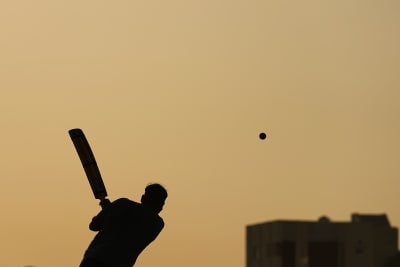A captivating sunset photograph captures the dramatic silhouette of a cricket player mid-swing, with his bat held aloft over his left shoulder. The sky is aglow with rich orange and yellow hues, providing a vivid backdrop that contrasts sharply with the black silhouettes. The cricket ball is airborne, frozen in motion near the center-right of the image. Dominating the bottom half of the frame, the player stands to the left, while the bottom right features the dark outline of a building, adding depth to the composition. The rectangular photo, slightly altered by camera filters to enhance the warm colors, effectively conveys the dynamism of the player and the tranquility of the setting sun.